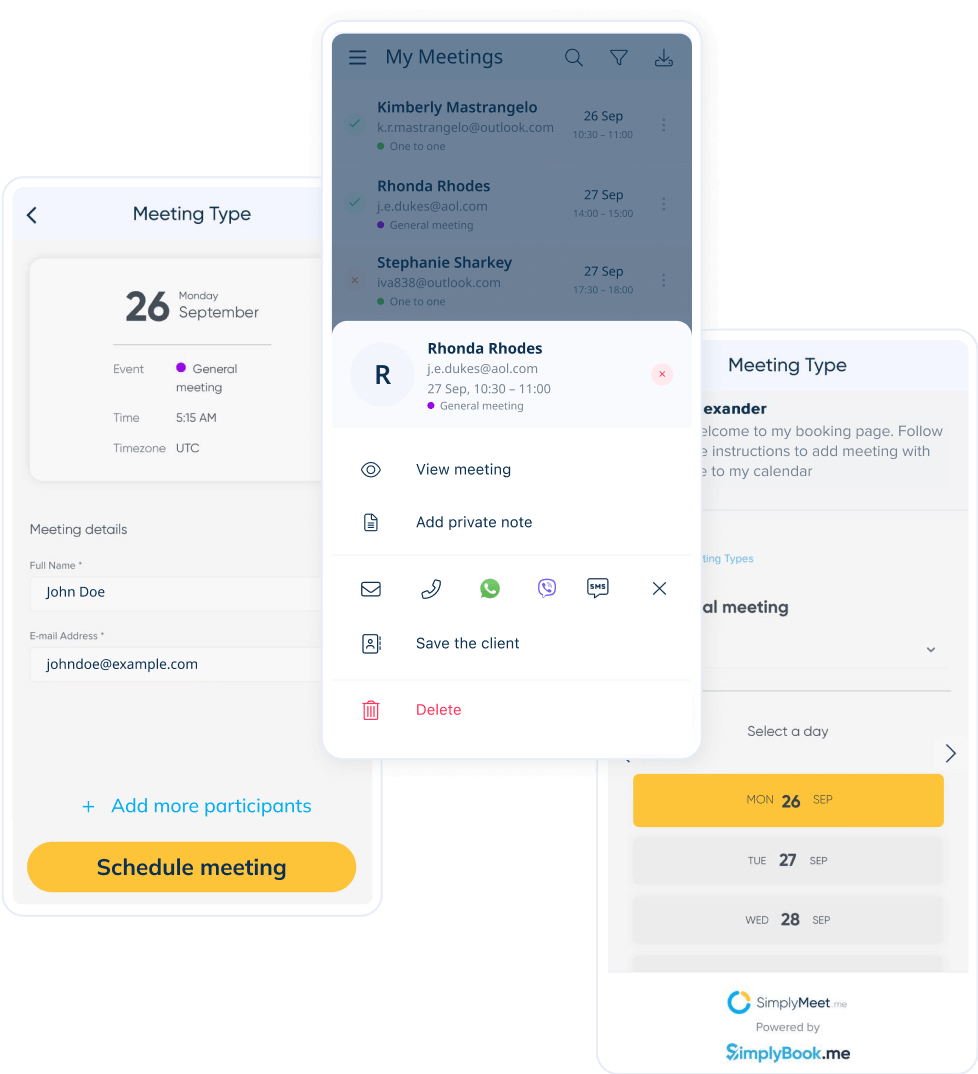The image features three overlapping screenshots from the same mobile phone app. The central screenshot is prominently displayed in the foreground, while two additional screenshots are partially visible behind it to the left and right, slightly lower in position. The central screenshot showcases an open app interface titled "My Meetings." A darkened background indicates that a pop-up prompt is taking precedence on the screen. The pop-up pertains to a meeting with Rhonda Rhodes and provides the following details: a web address, the meeting date and time (September 27th, 10:30-11:00 AM), and a description labeled "General Meeting." The prompt offers action buttons to view the meeting or add a private note, along with several icons for further actions such as email, text, or chat, represented by an envelope, a phone, and a chat bubble, respectively. The side screenshots depict different pages within the app, likely showing the interface one would use to set up a meeting.